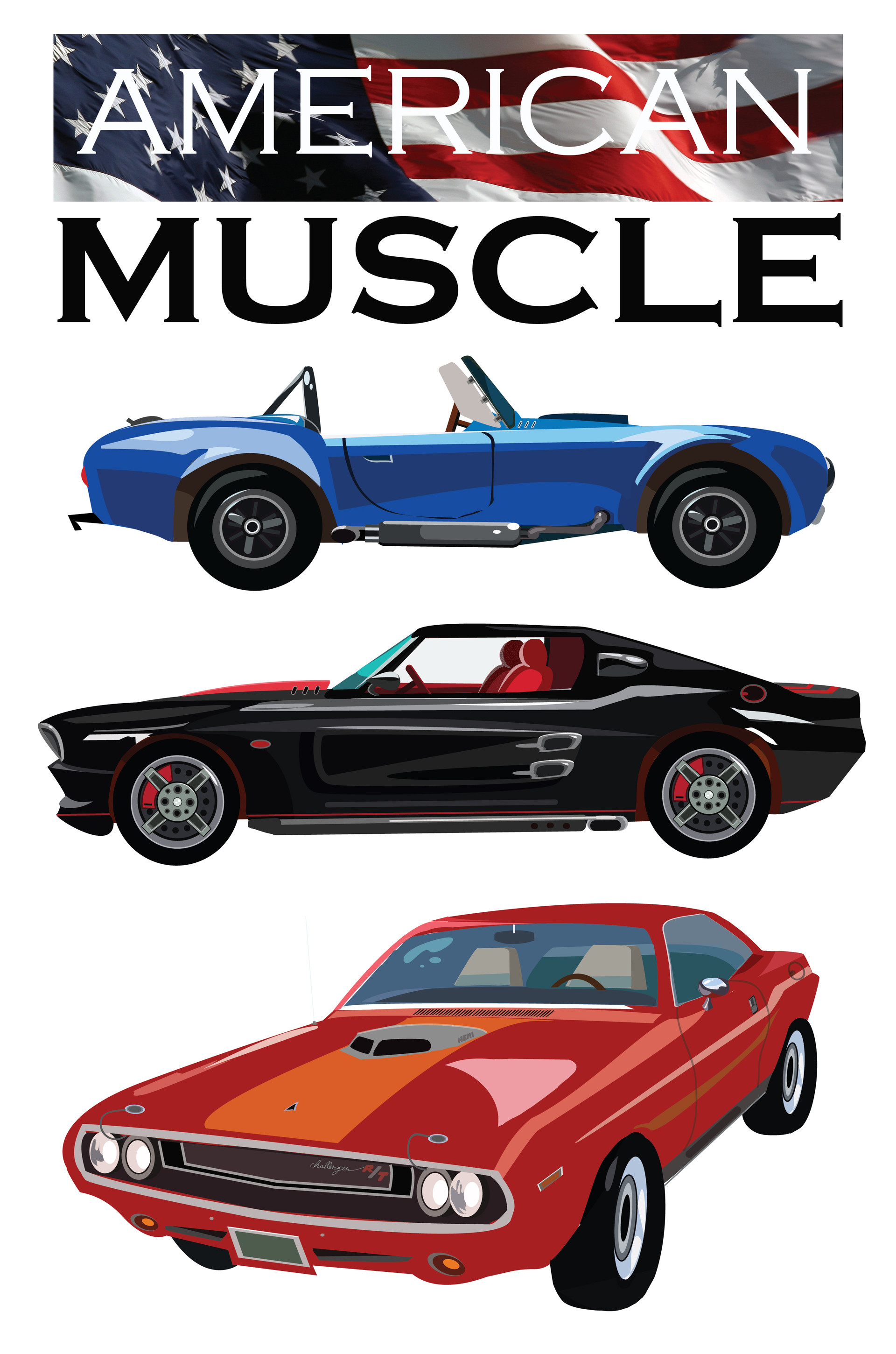This vibrant digital illustration features a series of vintage American muscle cars, stacked one above the other against a backdrop that prominently showcases an American flag at the top of the image. The text "AMERICAN" in bold white uppercase letters is emblazoned across the flag, followed by the word "muscle" in black beneath it. The first car in the series is a distinctive blue convertible with a roll bar at the back, reflecting classic automotive design. Below it, a sleek black hardtop, resembling a Mustang, is depicted with striking red interior accents. The final car in the sequence is a bold red muscle car, possibly a Camaro or Chevelle, with a notable feature on its roof, adding to its robust appearance. The colors in the image range from the patriotic red, white, and blue to the stark contrasts of black, gray, and orange, creating a dynamic and eye-catching composition likely intended for an advertisement.